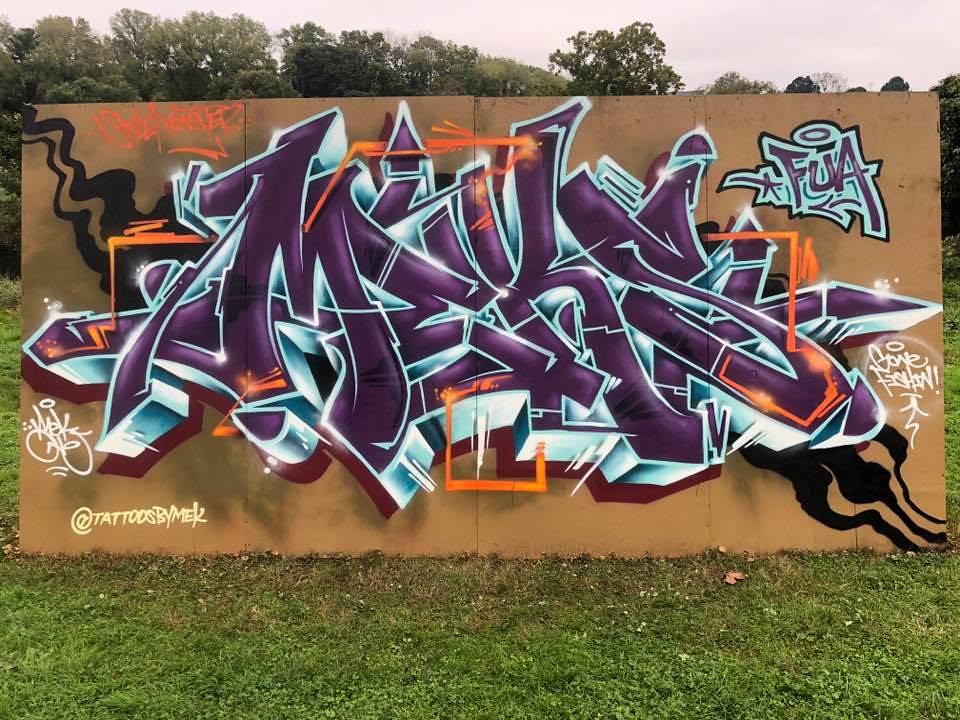The image features a detailed, vibrant graffiti artwork displayed on a makeshift wall constructed from four pieces of plywood, which are propped up on a bed of green grass. The graffiti comprises intricate, 3D-styled lettering with a striking metallic sheen, primarily in shades of purple, accented with white, orange, aqua blue, and black. Although the full text is not entirely legible, letters such as "M," "K," and possibly "S" can be discerned. Additionally, there is a smaller piece of graffiti in the top right corner spelling "F-U-A." At the bottom of the composition, the graffiti artist's tag reads "Tattoos by Mech" or "M-E-K." The scene is set outdoors during the day, with lush green trees visible in the background, creating a vivid and dynamic visual against the earthy backdrop.